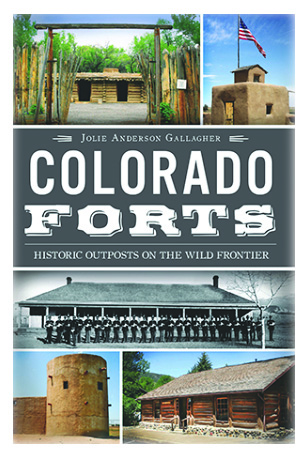This detailed, full-color magazine page prominently features "Colorado Forts: Historic Outposts on the Wild Frontier" by Jolie Anderson Gallagher. Centered on a gray background, the title divides the page where a black-and-white photograph lies, showcasing a long historical building with numerous soldiers standing in a row in front of it. 

At the top left, there's an image of a log cabin visible through a fence and an entryway constructed from tree posts. Adjacent to this, in the upper right, a fort appears made of mud, crowned with a United States flag on a flagpole. 

Towards the bottom of the page, the left side reveals a beige tower-like structure, possibly plastered or made of mud, while the bottom right features a large log cabin-like fort. These varied images collectively highlight the diverse construction styles of Colorado's historic forts.